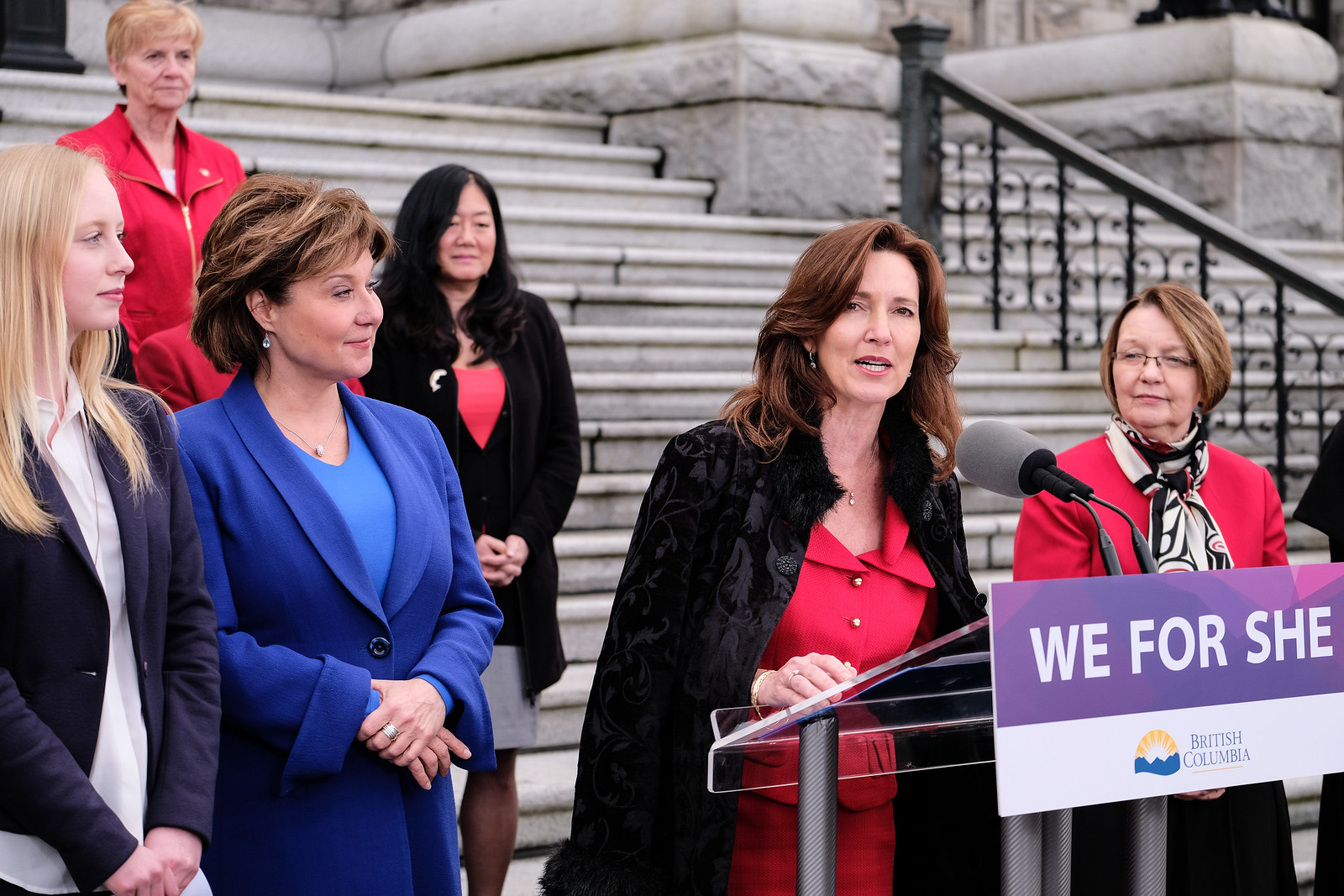This image captures a scene of a woman giving a speech at an event, presumably related to women's rights or advocacy. The woman stands behind a glass podium supported by metal poles, which prominently displays a purple sign that reads "We For She" in white lettering. Beneath this, the sign states "British Columbia" along with the province's logo showcasing mountains and a sun.

The speaker is dressed in a striking red outfit with a black coat draped over her shoulders, and she speaks into a large gray microphone. She has brown hair and her complexion is fair. The backdrop consists of a series of concrete steps ascending behind her, with a black railing visible to the right.

Surrounding the speaker are five other women, each attentively focused on her, smiling and seemingly proud. Their varied appearances are notable: one has short brown hair and wears a blue outfit; another has long blonde hair and is dressed in black and white; there is an older woman with blonde hair in red attire, an Asian woman in a combination of black and red, and another older woman with brown hair also dressed in red standing nearby. The diversity in their appearances and attire adds to the inclusive atmosphere of the gathering.